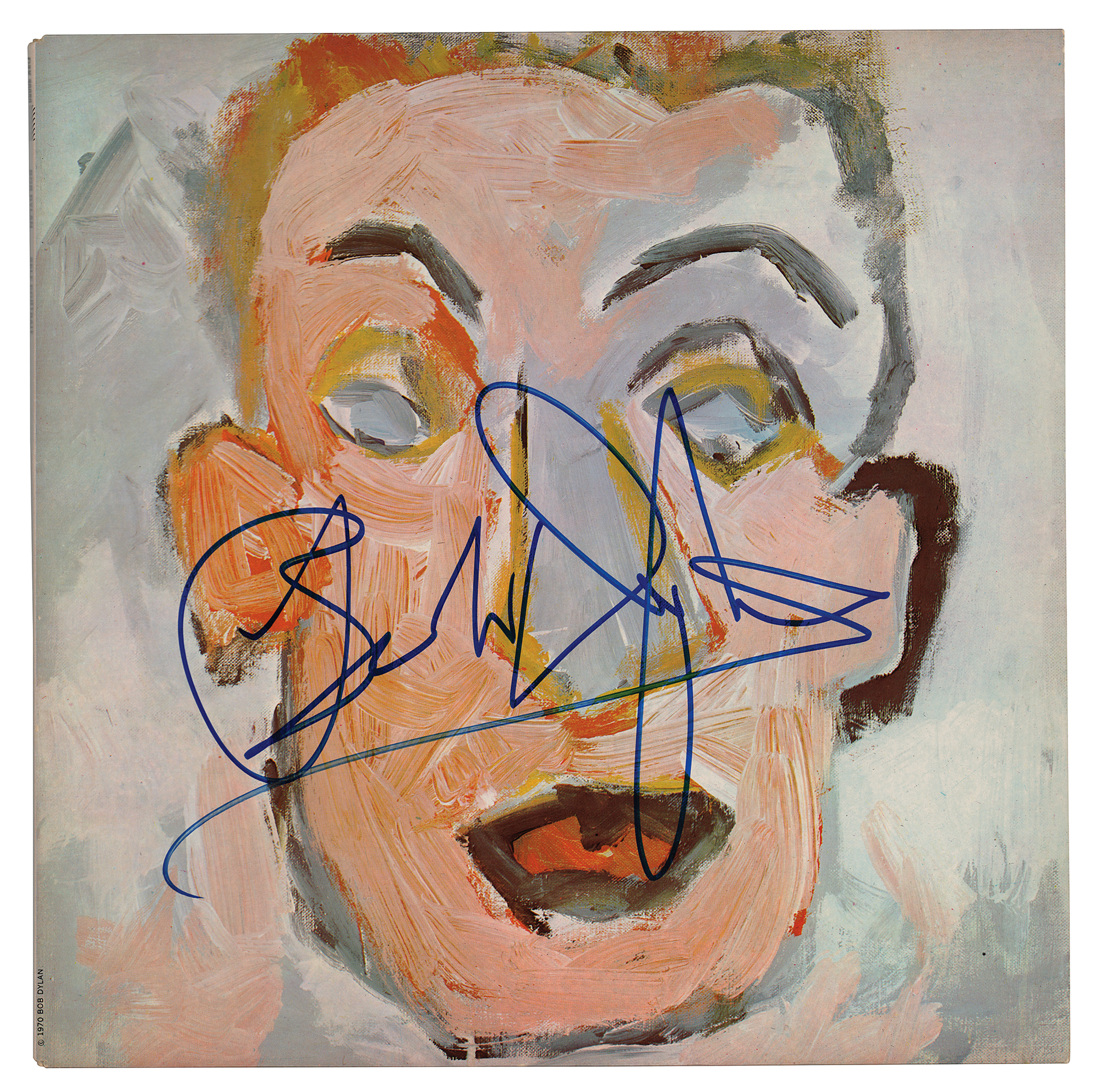This image features an abstract portrait likely created with oil pastels. At its center, it depicts a man's face characterized by exaggerated and surreal features. The face is predominantly orange with short, mustard-yellow hair. The eyes and nose are gray, with the nose appearing fairly large. The raised eyebrows are black, and the lips are a dark brown, with the mouth's interior shaded in darker orange. The man's ears stick out slightly, adding to the peculiar charm of the painting. Draped across the face in thin dark blue ink, there's a signature, which appears to read "Bob Dylan," and includes a "copyright 1970" mark, also by Bob Dylan. The background is composed of varying shades of gray, interspersed with patches of peach, white, and slight orangey-peach hues toward the bottom. This distinctive combination of colors and features gives the painting its unique, expressive quality.